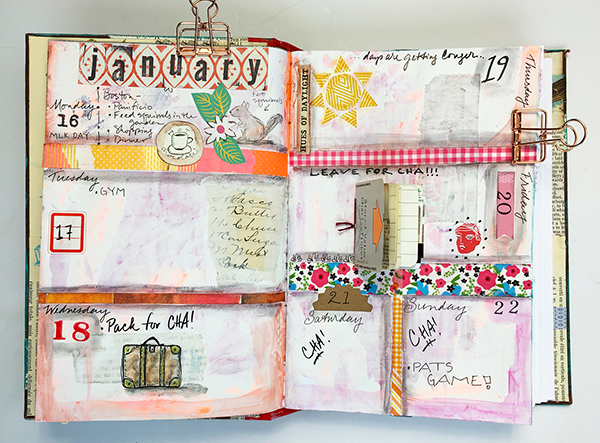This image features an open personal planner or diary, depicted in a book form, organized to display the week of Monday, January 16th through Sunday, January 22nd. Brass clips secure the pages at the top corners, making the entries clearly visible. The left page begins with "January" at the top, highlighting Monday the 16th as Martin Luther King Day, embellished with a drawing of a squirrel and mentions of feeding squirrels and a planned dinner. Tuesday the 17th simply notes "gym," while Wednesday the 18th instructs to "pack for CHA" with an illustration of a suitcase. The adjacent right page continues with Thursday the 19th, noting "days are getting longer" accompanied by a sun drawing or stamp. Friday the 20th includes a "leave for CHA" reminder with a head drawing. The weekend entries mark an eventful schedule: Saturday the 21st and Sunday the 22nd both denote "CHA," with Sunday additionally highlighting a "Pats game," likely referring to a New England Patriots football game.